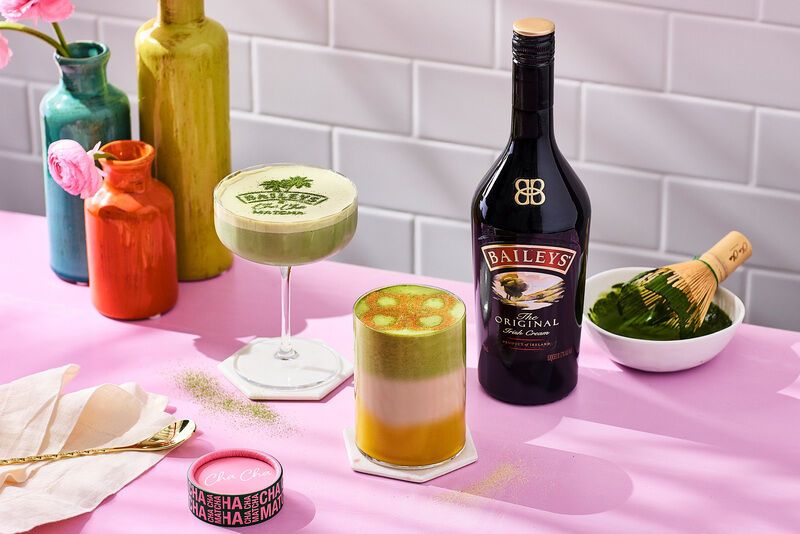This professionally-taken photograph features an elegantly arranged table set against a white brick wall backdrop, enhanced with fine grout lines that add texture to the scene. The table, draped in a pink tablecloth, showcases a variety of colorful and intriguing items. Dominating the right side is a full bottle of Bailey's Original Irish Cream, its iconic black bottle adorned with a gold cap and the distinctive Bailey's logo in red and gold lettering.

In the center foreground, a visually striking layered cocktail captivates with its vibrant hues: green foam crowns the top, beneath which lie layers of pink and yellow, accented further by orange and green dots. To its left, a martini glass filled with green liquid is decorated with edible writing on its white foam surface, showcasing the Bailey's logo in green.

Adjacent to these drinks, a small white bowl containing dark green matcha powder and paired with a wooden stirrer adds an exotic touch to the arrangement. Near this bowl, a round pink object inscribed with what seems to read "Ha-something" adds an element of curiosity.

To the left section of the table, three vases stand tall, each holding pink flowers with green stems. The vases differ in color: vibrant teal, rich red, and a golden hue, each adding to the composition's chromatic diversity. Resting on a beige napkin at the forefront is a delicate gold stirring spoon, completing the meticulously detailed setup.